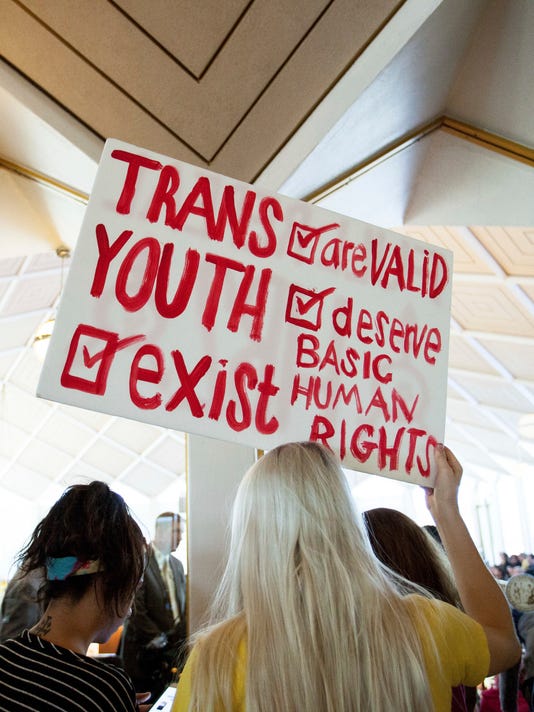The photograph captures a poignant and energetic protest for trans youth, set inside a building with a distinctive angled coffered ceiling, featuring light tan squares bordered in white. The room’s modern architectural lines add to the focused yet chaotic atmosphere as a sizable crowd fills the space, with many people either occupying or attempting to enter the room. At the center of the image stands a woman with long platinum blonde hair, clad in a yellow shirt, her back turned to the viewer. She is prominently holding up a white poster board with red handwritten font. The sign reads: "Trans [check mark box] are valid. Youth [check mark box] deserve basic human rights. [Check mark box] exist." Next to her, a woman with dark hair, a striped shirt, and a headband also faces away from the camera, adding to the scene's depth and intensity.